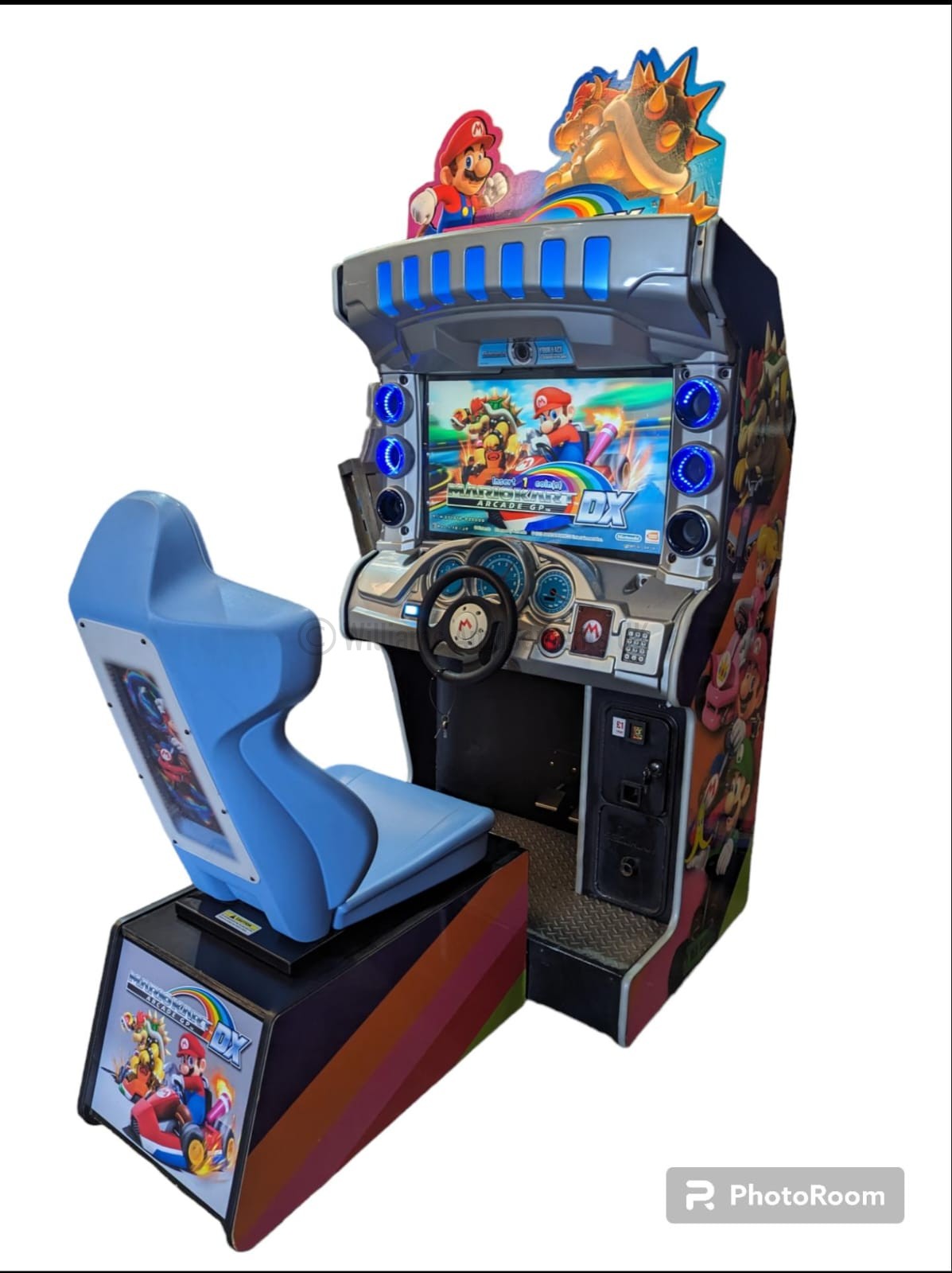The image depicts an arcade game setup featuring the well-known Super Mario Kart racing experience. The tall and imposing arcade cabinet boasts a large widescreen display encased in a sleek silver frame, accentuated with glowing blue LED strips which run along the sides and top, adding a modern touch to its appearance. At the pinnacle of the cabinet, a vibrant sign showcases a rainbow background with Mario on one side and a dinosaur character, likely Koopa, on the other, suggesting a thrilling racing duel.

Beneath the screen, there is a steering wheel attachment flanked by blue-colored speedometers and various buttons, providing a hands-on, immersive experience. A coin slot is also visible at the bottom, essential for starting the game. The prominent black line borders the bottom, right, and top edges of the display, and in the bottom right corner, a gray rectangle logo with white text reads "Photo Room." 

Adjacent to this logo is a P&R emblem. The large, molded seat is a striking light blue, attached to a solid black metal base, designed for comfort and stability during gameplay. A sticker adorns the back of the seat. The chair and steering setup is complemented by a distinctive box, featuring black, orange, pink, red, and green stripes.

Overall, the detailed elements, from the dynamic on-screen Mario Kart DX title to the rainbow-themed top sign with beloved characters, all come together to make this arcade unit an eye-catching and engaging attraction for gaming enthusiasts.